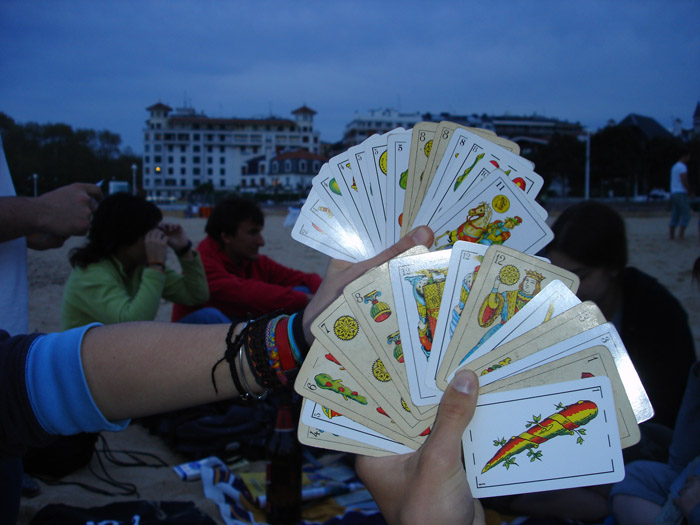A close-up captures a group of people seated in a sandy, open area as dusk approaches. The dim light casts a soft glow on tall, white buildings and the silhouettes of trees in the background. In the mid-ground, a woman wearing a green sweater sits next to a man in a red sweater, partially illuminated by the fading light. In the foreground, the detailed focus shifts to two hands holding fanned-out cards. The left hand, adorned with numerous colorful bangles, belongs to a person wearing a black and blue sleeve. The second hand, only visible as a left hand, also holds a fanned arrangement of cards, contributing to the intimate and serene ambiance of the evening scene.